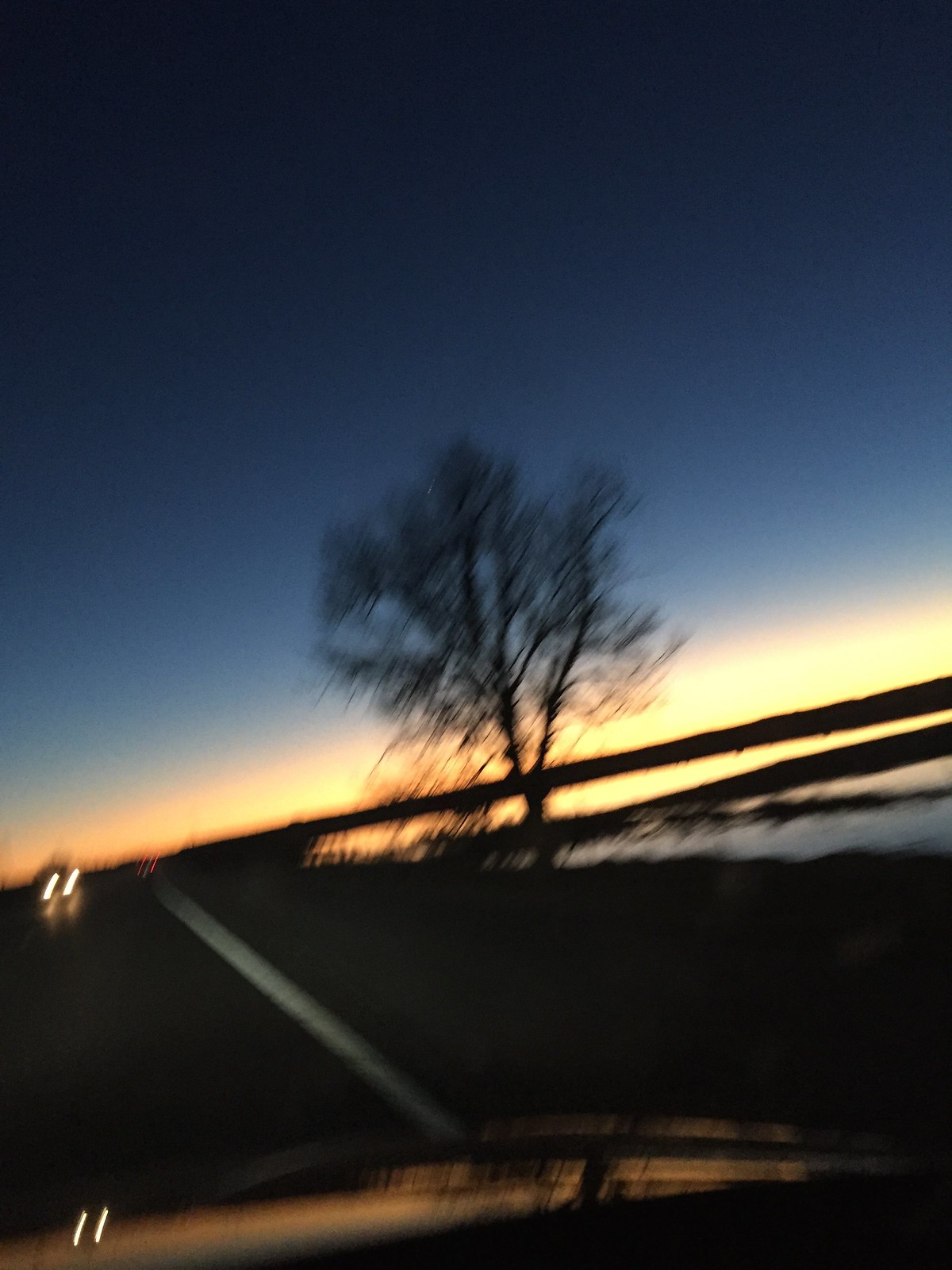In this vertically oriented photograph, we are presented with a scene of a captivating, albeit blurry, sunset. The image is framed by a wooden fence in the foreground, which separates the viewer from a road where a car with its headlights on is traveling westward. Central to the composition is a solitary, leafless tree standing stark against the landscape.

Beyond the road lies a snowbank, indicating a wintry setting. Beneath this area, a brook or narrow river reflects the overall serenity, likely running underneath an overpass not visible in this frame. The sky is a gradient masterpiece, starting at the horizon with a radiant yellow that melds into a soft pink glow, transitioning into a light gray, which gradually darkens towards the top of the photograph. This blend of colors, despite the blurriness, lends a dreamy and tranquil aura to the scene.